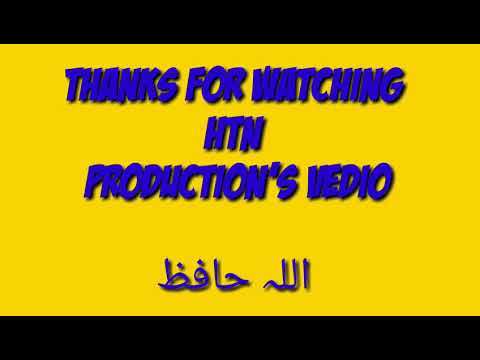The image features a yellow rectangular background bordered by black bars at the top and bottom. In the center, bold electric blue block letters spell out "thanks for watching HTN Productions VEDIO" along the top of the yellow area. The blue text is somewhat pixelated and has black specks and outlines, giving it a shadowy effect that stands out against the yellow. Below this text, there are characters in a foreign language, possibly Arabic or Hindi, also in blue and showing notable pixelation, especially around the edges.